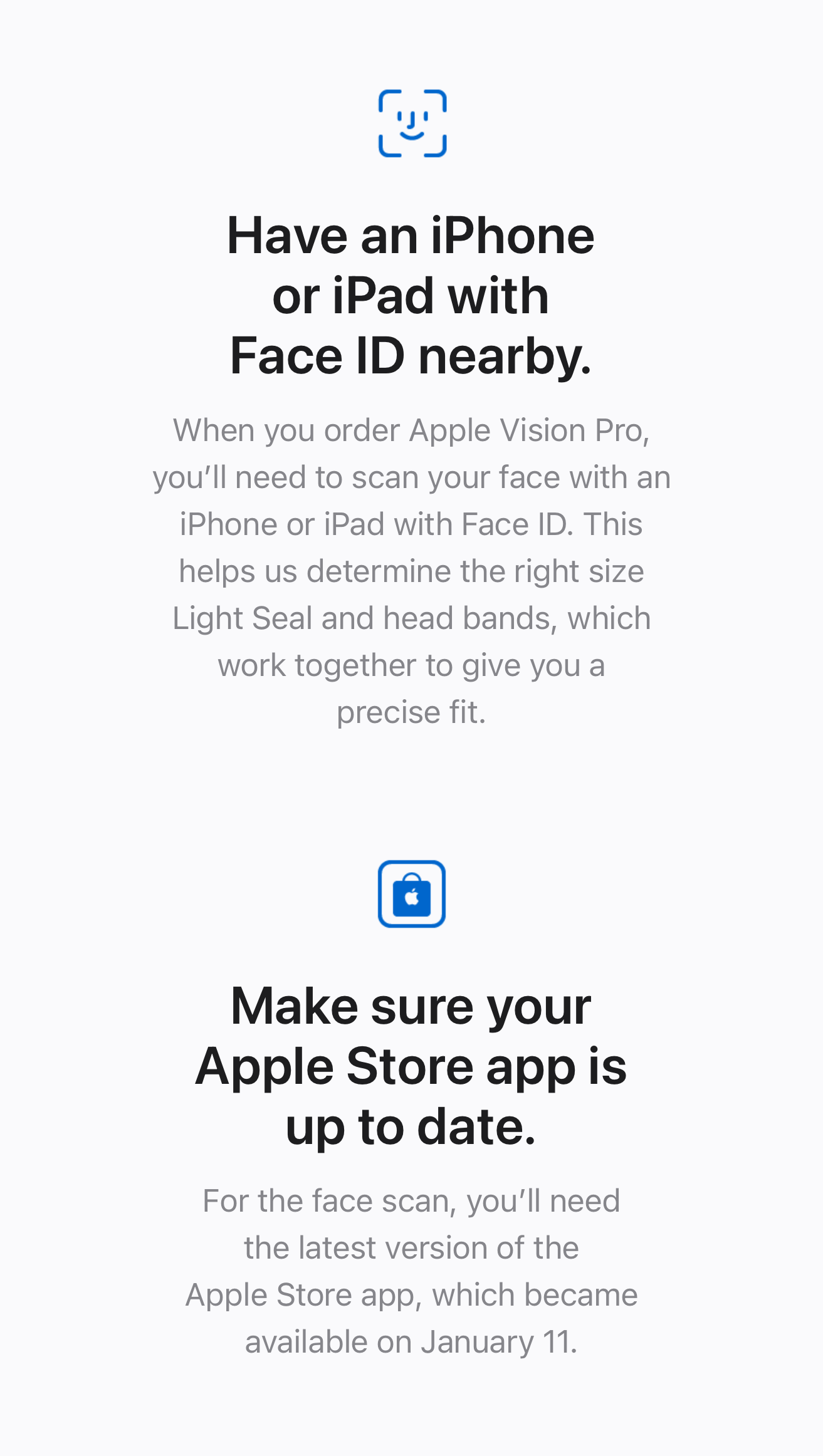Certainly! Here's a detailed and cleaned-up caption for the described image:

---

This screenshot showcases a web page with a light gray background and black text, divided into two sections. The top section features a title, "Have an iPhone or an iPad with Face ID nearby," accompanied by an icon of a smiley face. Below the title, a description reads, "When you order Apple Vision Pro, you'll need to scan your face with an iPhone or an iPad with Face ID. This helps us determine the right size, light seal, and headbands which work together to give you a precise fit."

The bottom section is titled "Make sure your Apple Store app is up to date," featuring an icon of a shopping bag with the Apple logo. The following text states, "For the face scan, you'll need the latest version of the Apple Store app, which becomes available on January 11th." The layout is simple and primarily provides essential information for users ordering the Apple Vision Pro.

---

This caption elaborates on each visual and textual component of the image, ensuring clarity and detail.